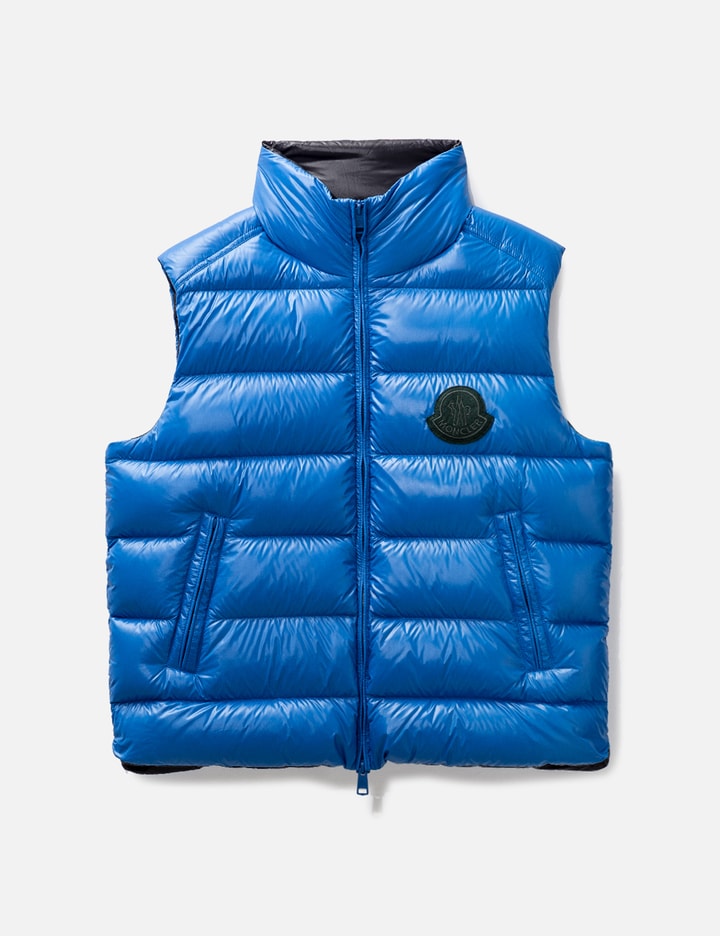The image features a bright royal blue down vest set against a white background. The vest has a highly puffy appearance, indicative of its down filling, which is arranged in seven horizontal padded bands running vertically down the garment. It features a high collar that zips all the way up the neck, with a blue zipper centrally located. The interior of the collar is lined with a glossy black fabric, adding a sleek contrast to the vest’s exterior material, which appears to have a plastic gloss or PVC finish.

The vest is notable for its two diagonally set front pockets, and a circular brown emblem with an indiscernible brand name on the left side (from the viewer's perspective), adding a touch of detail to the design. It's not possible to determine the vest's size or intended wearer from the image alone, as there are no size indicators or models wearing it. The vest is displayed alone, emphasizing its features and its vibrant color.